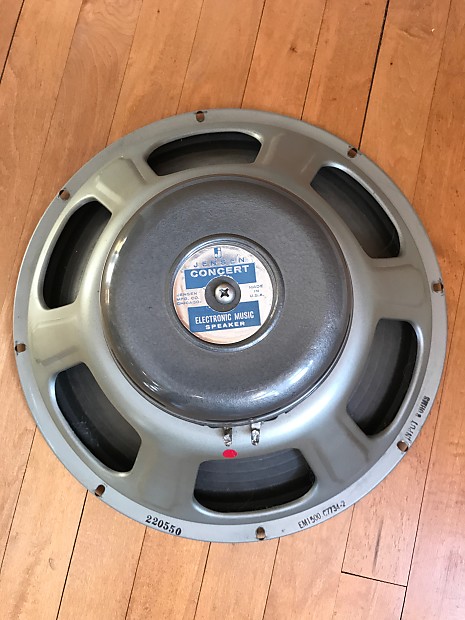This detailed overhead photograph captures a round, metal car speaker, approximately 12 to 15 inches in diameter, lying face down on a medium-brown wooden floor with slats running vertically. The speaker, which appears to be from a brand called "Jensen," has a light silver, coned-up edge with eight screw holes evenly spaced around it. Around the circumference, there are two-inch wide and long grooves designed for air circulation. The main body is dark gray, and at its center is a white circle featuring two blue boxes with the text "concert" and "electronic music speaker" in white. The blue boxes are separated by a central screw. Also visible are various serial numbers, including "220 550," and the phrase "Made in the USA" stamped on the back.